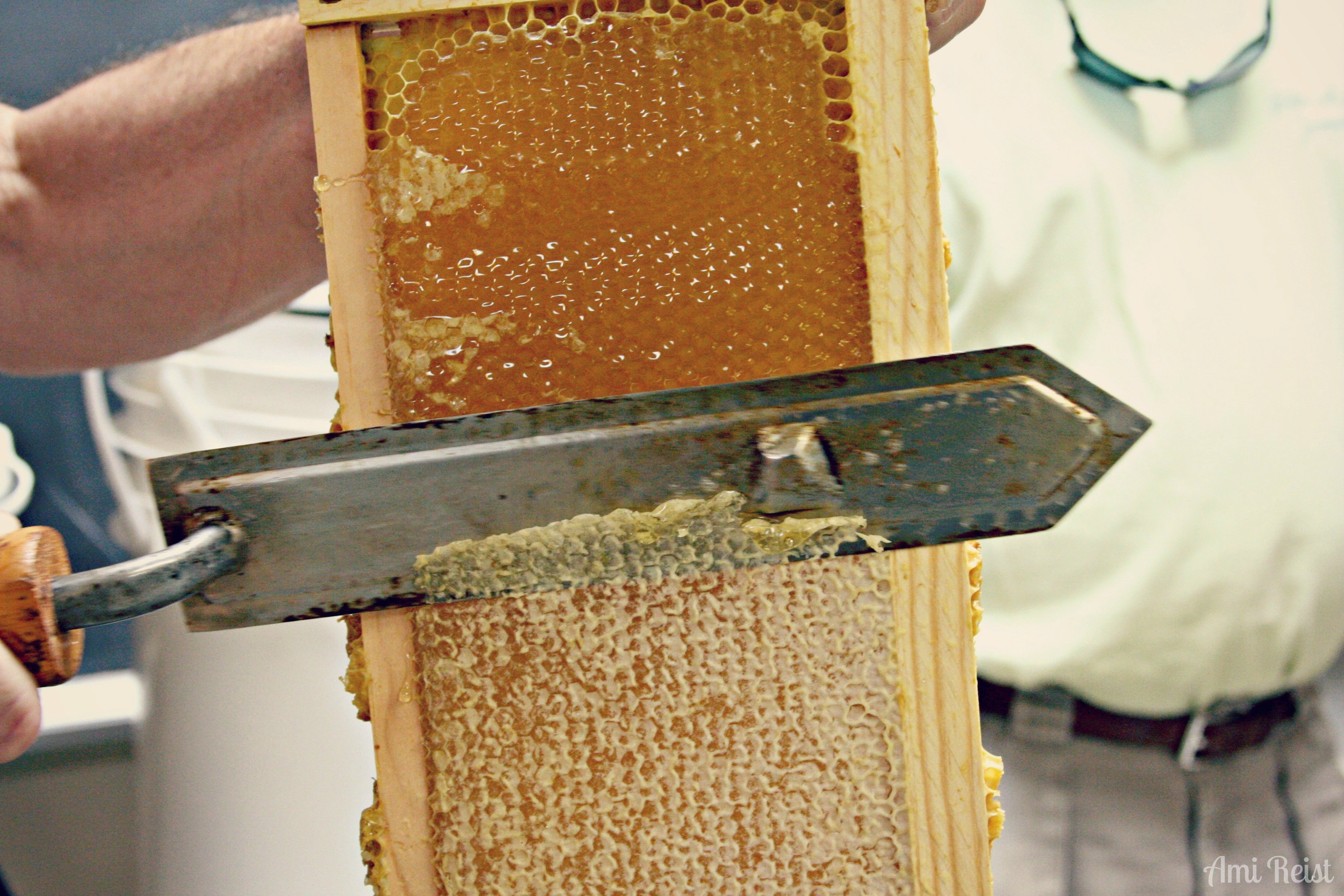The photograph depicts a close-up of a rectangular wooden frame filled with honeycomb, freshly pulled out of a beehive. The honeycomb is the central focus, showcased in a rough wooden frame, filled with golden honey and capped beeswax. Just above the honeycomb, someone’s blurred silhouette in a white shirt and gray pants appears in the background, with sunglasses hanging from their neck. Their forearm extends into the foreground holding the honeycomb, while their other hand wields a broad, iron-like tool, typically used by beekeepers. The tool is actively shaving or melting off the wax cappings from the cells, revealing the shiny, amber honey beneath. The top part of the honeycomb glistens where it has been uncapped, contrasting with the lower section which retains its waxy appearance. Another person's torso is partially visible on the right side of the image, observing this meticulous process.